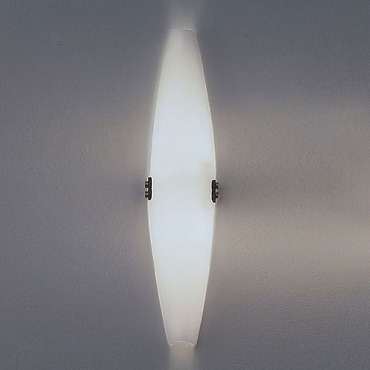The image is a striking black-and-white photograph in a square format, featuring a futuristic and minimalistic central object. This object, which could be a light or a vase, is tall and cylindrical, narrow at both the top and bottom while expanding toward the middle, creating a symmetric and elegant form. The surface of the object appears translucent and white, radiating a soft glow that suggests it might be illuminated from within. On either side of the glowing cylinder, precisely in its middle section, are two small black attachments that resemble Lego pieces or hinges. 

The background of the image is a dark gray gradient, shimmering and slightly out of focus, which adds to the modernistic and ethereal feel of the composition. The light from the central object softly reflects on the background, creating warmer, lighter zones near the center while leaving the edges in a darker gray shade. This gradient effect enhances the overall impression of a light-colored opening in a dark, almost silvery void, embodying a style of photographic realism.